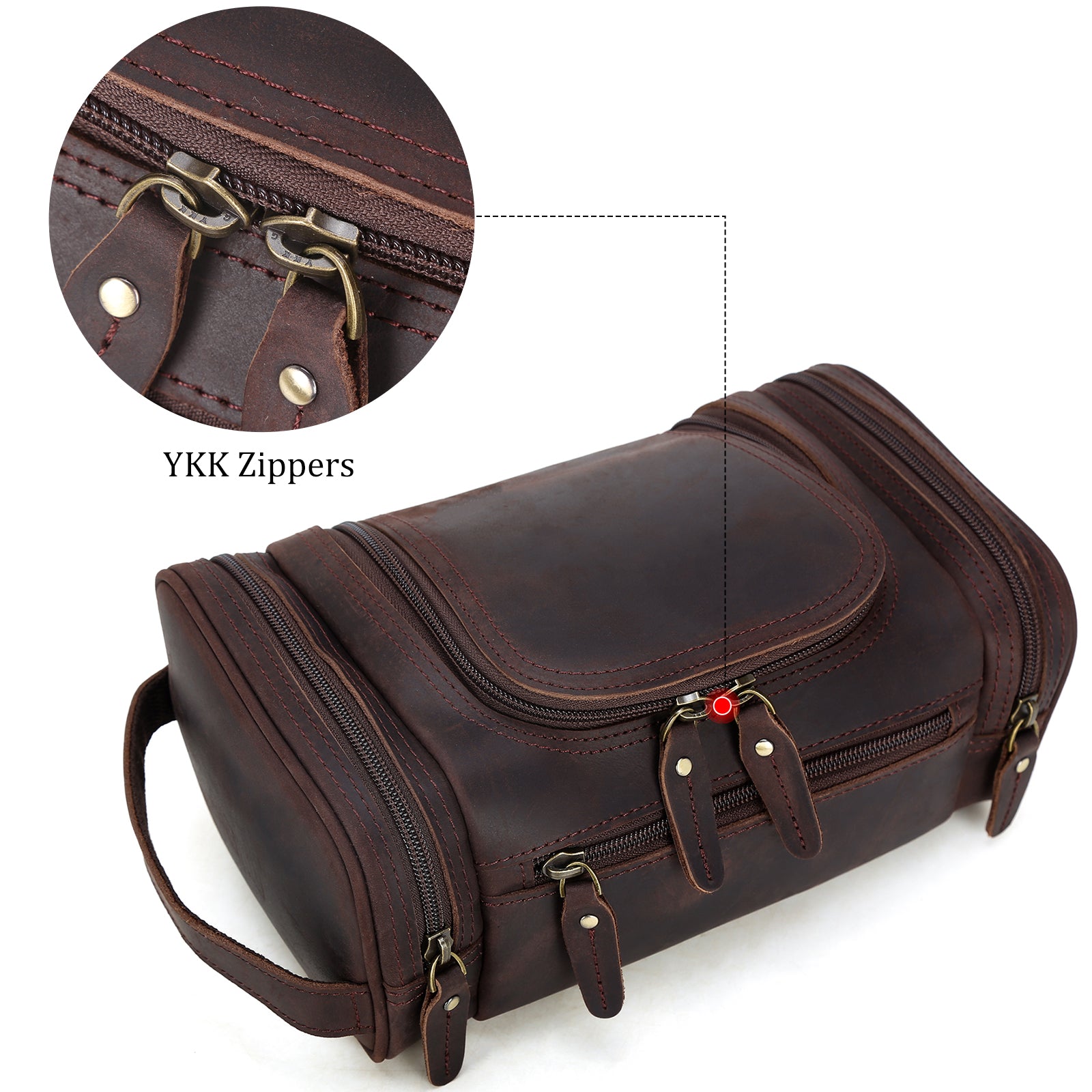The image showcases a large, dark brown leather bag, possibly a duffel bag or suitcase, prominently featuring numerous zippers. The bag has a cylindrical, slightly rectangular shape with lighter brown accents outlining the zippers and edges. A sturdy handle is situated at the top of the bag. In the top left corner of the image, there's a circular inset containing a close-up of two zippers, highlighting their detailed construction. A dotted line connects this inset to the bag, emphasizing the zippers. Below the inset, the text "YKK Zippers" is visible, indicating the brand of the zippers. The entire advertisement is set against a bright, well-lit white background, enhancing the clarity and prominence of the bag's features.